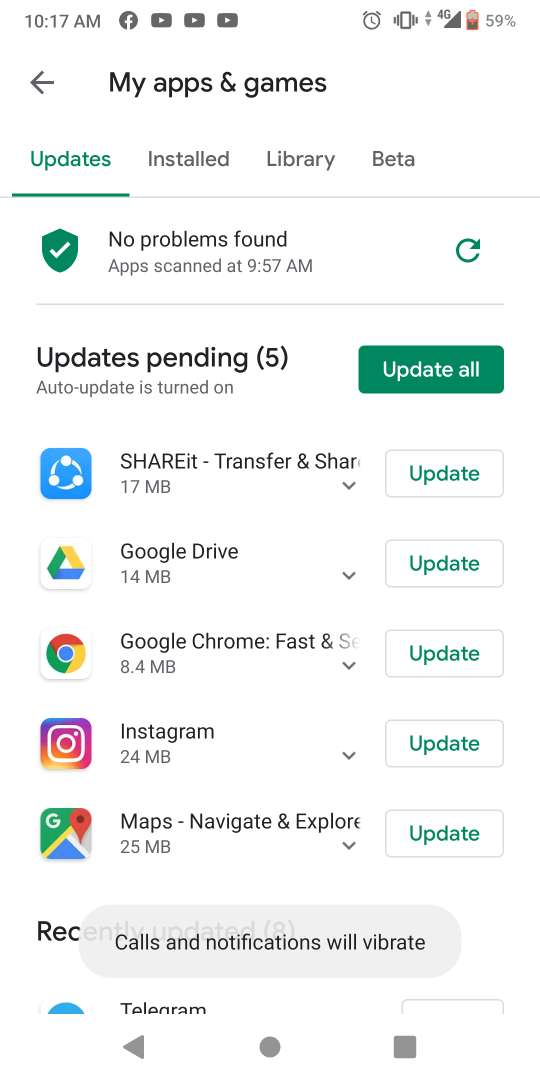The screenshot, captured on a cell phone, displays the "My Apps & Games" section of the Google Play Store. In the top left corner, the time is shown to be 10:17 AM, while the top right corner indicates the battery level at 59%. The screen is specifically focused on the "Updates" tab, one of the four options available beneath the page title, the others being Installed, Library, and Beta.

The image details five pending application updates listed in a vertical arrangement:
1. Share It
2. Google Drive
3. Google Chrome
4. Instagram
5. Maps

Next to each application name is an "Update" button, and above this list is an "Update All" button for convenience. The background of the page is entirely white, creating a clean and straightforward interface for the user.